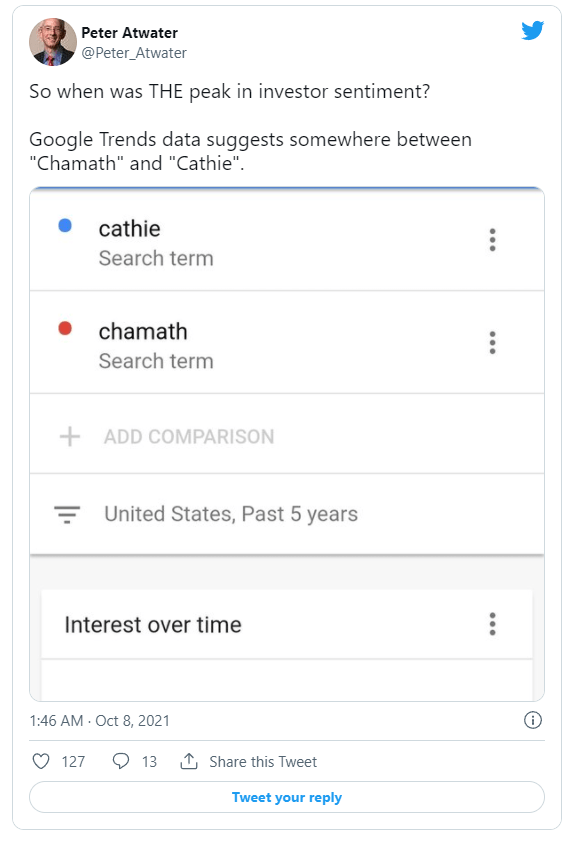This is a screenshot of a Tweet by Peter Atwater, whose handle is @Peter_Atwater. At the top right corner of the Tweet, the blue Twitter logo is visible. The tweet reads: "So when was the peak in investor sentiment? Google Trends data suggests somewhere between 'Chamath' and 'ARK Invest'." 

The image shows a comparison chart with 'ARK Invest' highlighted in a blue circle on the left as a search term, and 'Chamath' highlighted in a red circle below it as another search term. Beneath these, there is an option to add another comparison. The chart spans data from the United States over the past five years, illustrated with three horizontal bars, presumably representing search interest over time.